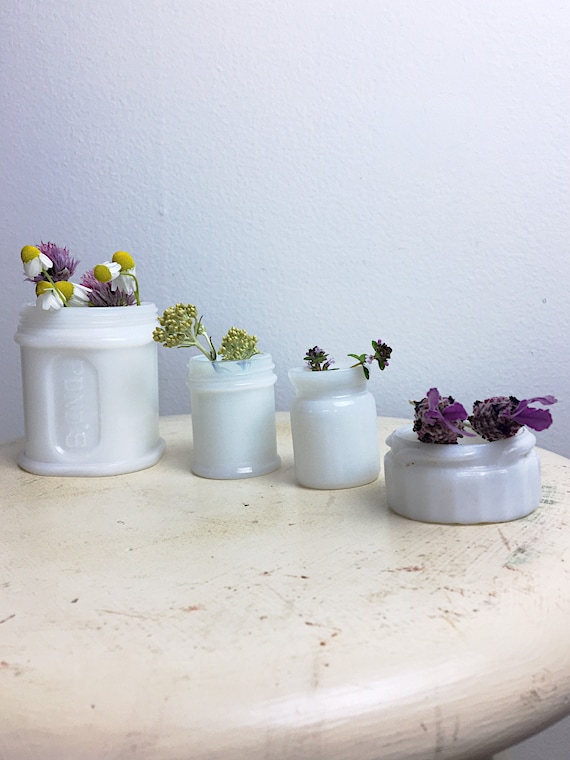This indoor color photo captures a well-worn, circular beige wooden table positioned against an off-white wall. The table surface is noticeably scuffed, indicating extensive use. Atop the table, there are four white containers, each varying in size and height. The tallest vase, situated on the far left, appears to be a white milk glass vessel holding a mix of small white flowers with yellow centers and a couple of purple blooms, likely daisies. To its right, a shorter white milk glass vase contains light green flowers. The next vase is also made of white milk glass, slightly shorter and thicker than the second, and holds more purple flowers. Finally, the shortest and stoutest container on the far right, possibly another milk glass piece, features purple flower bulbs. The arrangement and condition of these flowers suggest they are being dried.